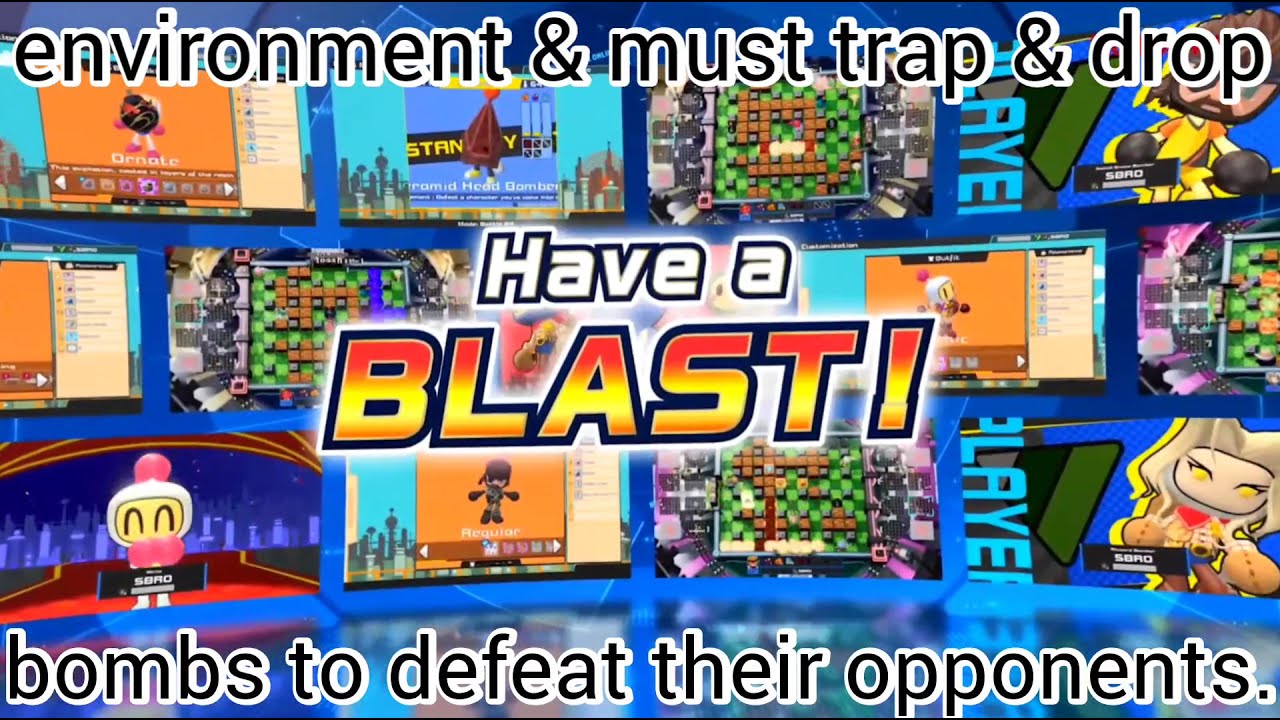The image is a dynamic and vibrant collage featuring 14 different screenshots from various levels and scenes of the Bomberman video game series, arranged in three rows—four screenshots on the top row, six in the middle row, and four on the bottom row. Each screen showcases different characters, mazes, and explosions typical of the Bomberman franchise, with diverse colors including blue, orange, green, pink, and purple. 

At the forefront, in large, eye-catching text, it says "Have a blast!" The text "have a" is on the first line, and "blast!" is in a larger font with a gradient of orange, yellow, and dark orange colors, concluding with an exclamation mark. Below this, in smaller text, it reads "Bombs to defeat their opponents," hinting at the game's core mechanics.

The background screenshots show varied elements: the top row features an orange screen with a bomb creature, a partially obscured blue text possibly saying "Stanley," an intricate maze with strategically placed bombs, and a character with bomb hands and a bushy beard. Most of the middle row screens are concealed by the primary text, with minor variations among them. The bottom row includes a character with happy, expressive eyes and a pink hat and another screen depicted with a female character.

Surrounding the main image text, additional phrases like "environment" and "must trap and drop" suggest gameplay strategies. This richly colored and layered image appears to be an advertisement, possibly for a newer version of Bomberman, similar to what might be found on the back of a video game case or within a promotional showcase.